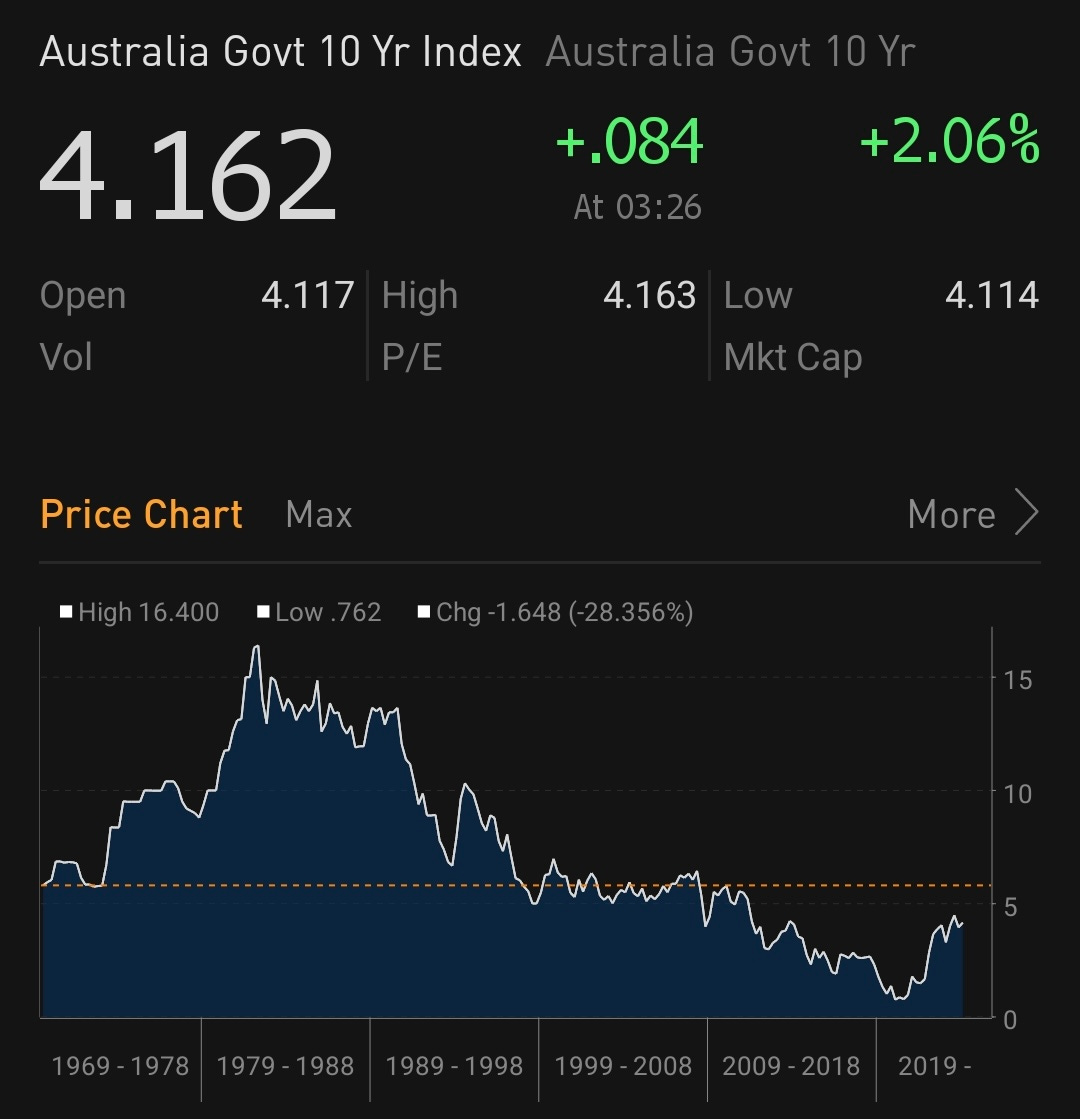This image is a screenshot, possibly a smaller segment of a screen from either a computer or a smartphone, featuring a dark, black background. At the top, the headline is prominently displayed in white font, reading "Australia GOVT 10-Year Index," followed by a secondary description in gray text, "Australia Government 10-Year," indicating it's related to bonds. Below the headline, the price is listed as $4.162 in white text, with a green font showing a positive change of +0.084. Further to the right, an additional increase is noted as +2.06%.

Underneath these figures, an orange title reads "Price Chart," introducing a detailed graph of price changes. The chart's line, depicted in blue, traces the price fluctuations from the year 1969 to 2019. Over this extensive timeline, the overall trend is downward, reaching a low in early 2019 before showing signs of recovery.